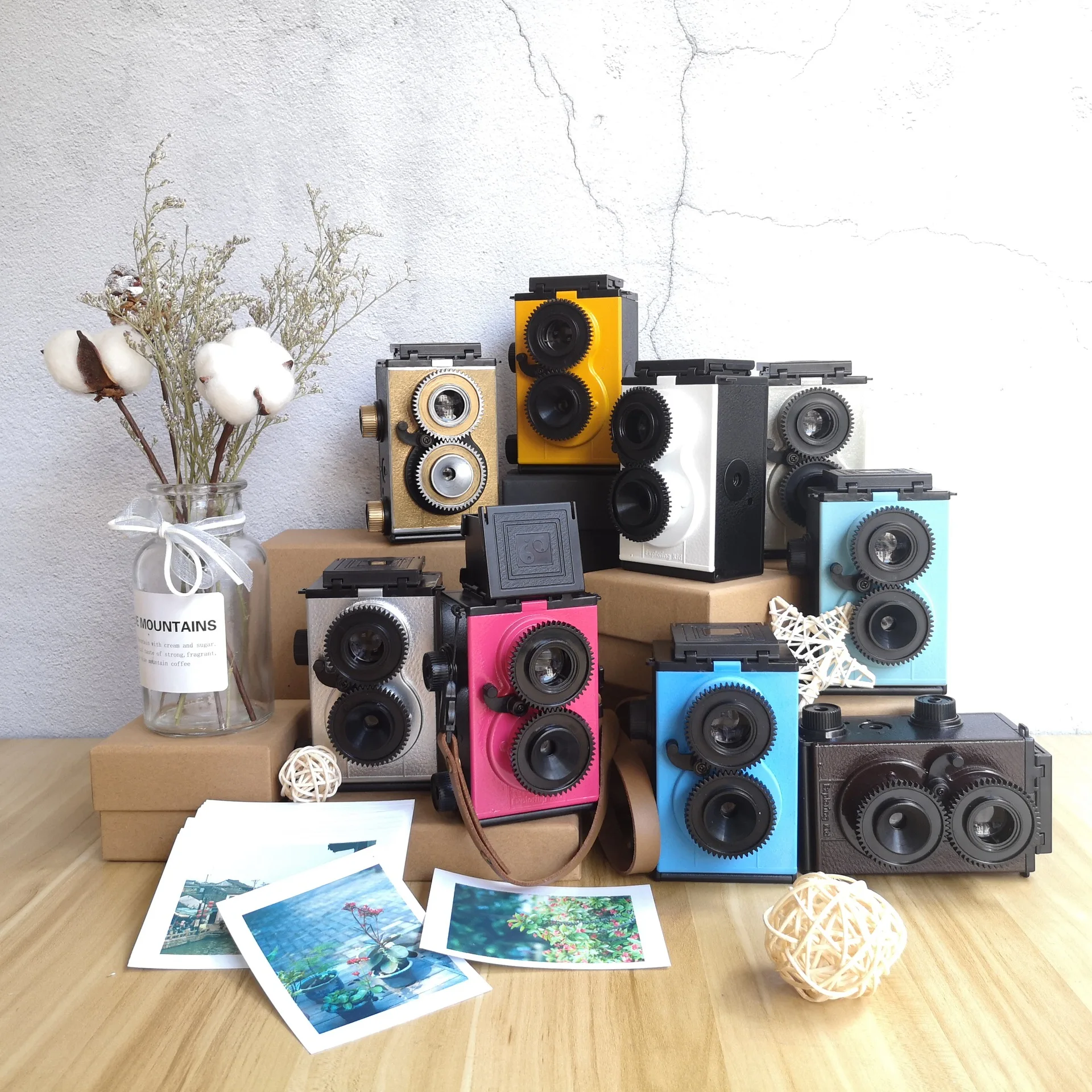The image showcases a collection of nine cameras, each adorned in a vibrant variety of colors including gold, yellow, white, blue, black, pink, and silver, displayed on what appears to be a beige bamboo tabletop. The cameras exhibit a modern take on vintage brownie-style designs, featuring multiple lenses, knobs, and folding viewfinders. The front of each camera is distinguished by colorful facades, such as turquoise, pink, yellow, ivory, and tan, giving the scene a lively and eclectic feel. To the left of the cameras, there's a clear vase filled with white flowers and dried baby's breath, adding a touch of elegance to the setting. On the floor in front of the cameras lie several Polaroid or printed photos, likely taken by these cameras. Additionally, a ball of white twine or string art is positioned prominently in the scene. The background wall is a simple white, ensuring that the colorful array of cameras and accessories remains the focal point.